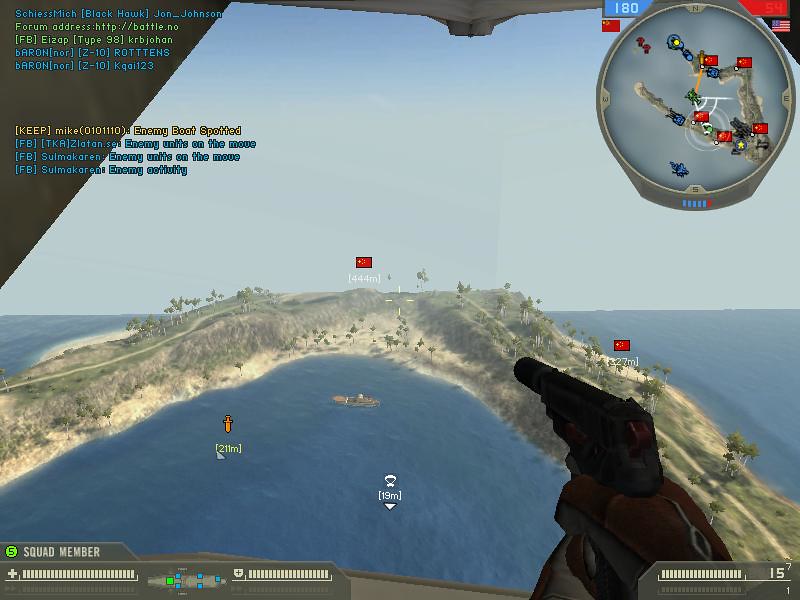The image depicts a scene from a video game set in a tropical, oceanic environment. In the bottom right-hand corner, a player is visible holding a handgun aimed towards various targets dispersed across the scene. These targets, some positioned on small boats and others floating in the open ocean, display the potential points to be earned when successfully hit. Additionally, a small stretch of land adorned with palm trees can be noted in the distance, adding a touch of greenery to the otherwise blue expanse. The clear blue sky overhead enhances the serene yet engaging atmosphere of the game. The interface reveals that the player, referred to as a squad member, has currently accumulated 15 points.